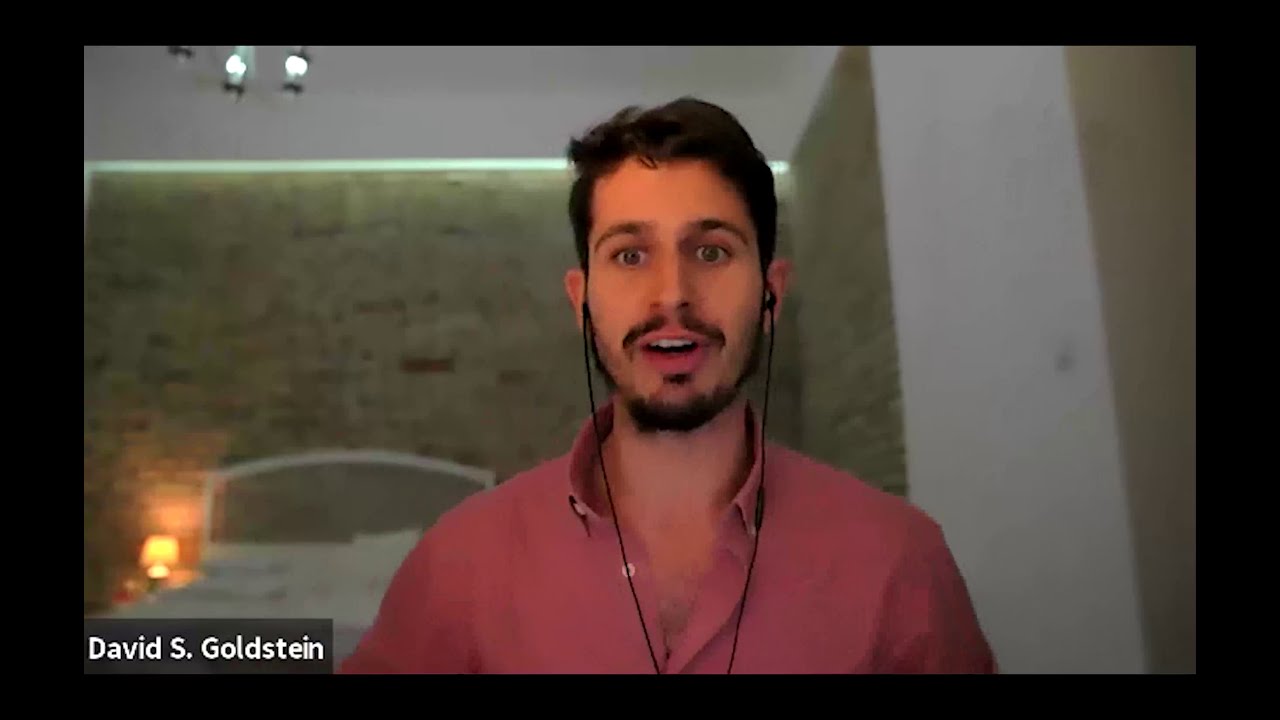The image is a screenshot from a video conference call featuring a man named David S. Goldstein, as indicated by the white lettering in a gray box in the bottom left corner. David is seated in what appears to be a bedroom or hotel room. He has dark, somewhat fluffy brown hair, a scruffy beard, a mustache, and brown facial hair. His wide eyes and slightly open mouth give him a surprised expression. He is wearing black wired earbuds and a salmon-colored button-up dress shirt that is open at the top, revealing part of his neck and chest. 

In the background, the room features tall brick walls in a tan or grayish color, a bed with white linens, and a headboard upholstered in gray and white. There is a lamp situated in the distance, and some ceiling lights are visible. A white door is positioned to his right. The entire image is bordered in black, adding a frame to the scene.